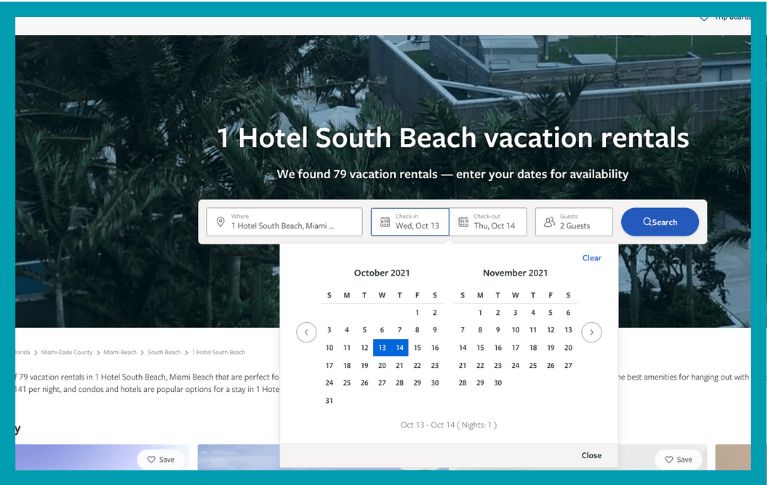Here is a cleaned-up and detailed caption:

---

This image is a screenshot bordered with a turquoise-colored frame. The background features a somewhat obscured aerial shot of a building surrounded by numerous palm trees. The screenshot showcases the search results page for "One Hotel, South Beach, Vacation Rentals," indicating that 79 vacation rentals have been found. Users are prompted to enter their dates for availability at "One Hotel, South Beach, Miami." The displayed check-in date is Wednesday, October 13, and the check-out date is Thursday, October 14, for two guests.

A calendar below this information shows the months of October 2021 and November 2021, with October 13 and 14 highlighted in a dark blue rectangle. No other dates are selected. The top right of the calendar section has a "Clear" option, and the bottom displays the range "October 13 through October 19" with "Nights one" and a "Close" option. 

To the left of the calendar, partially obscured text reads, "79 vacation rentals in One Hotel, South Beach, Miami Beach, that are perfect for [...]" and mentions that "per night and condos and hotels are popular options for a stay in One Hotel." The remaining text is blocked. On the right side, legible text includes "Best amenities for hanging out with [...]". 

At the very bottom of the screenshot, there is a white "Save" button with a black outlined heart next to the word "Save."